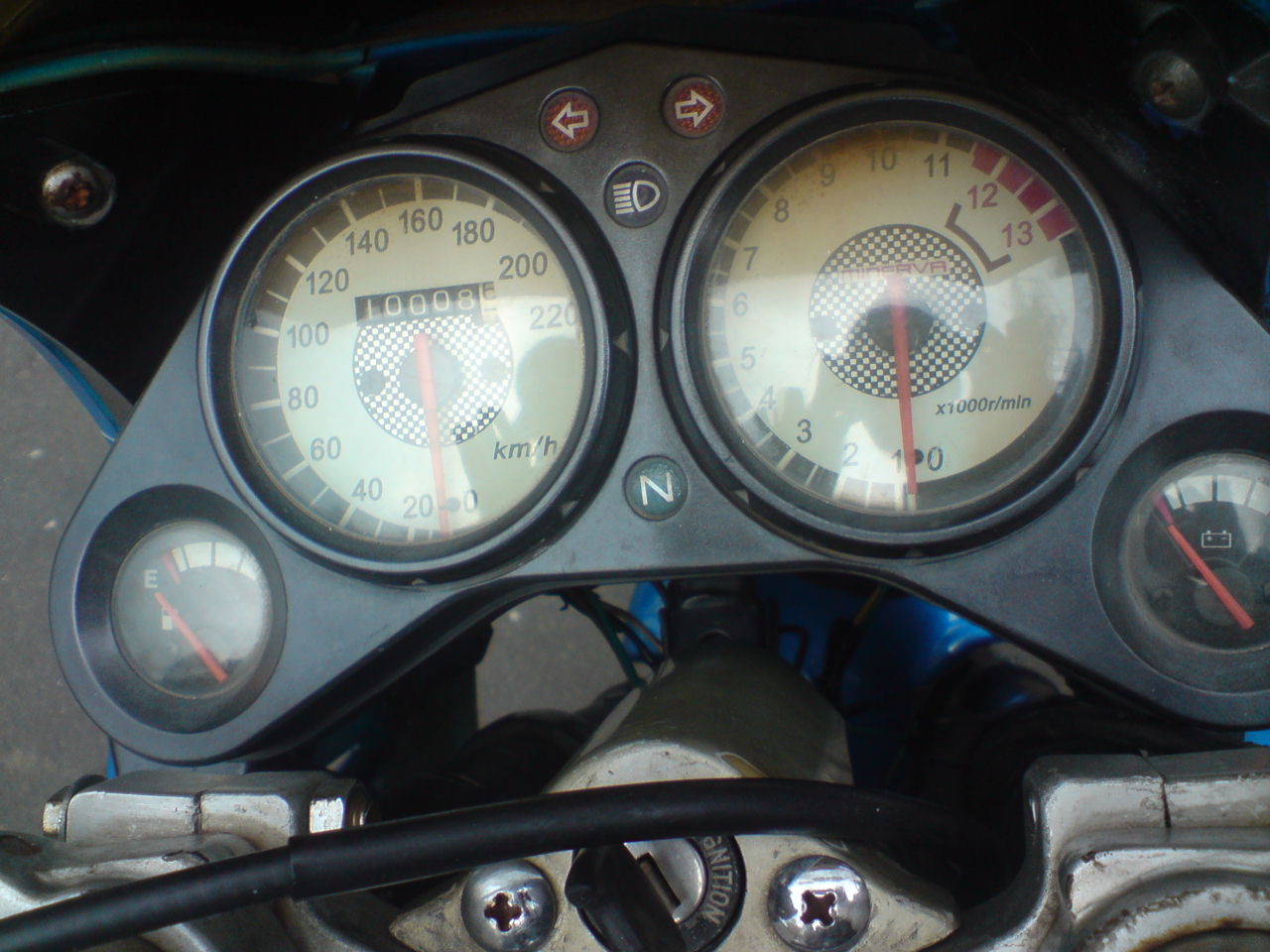A top-down view of a motorcycle's gauge cluster, showcasing its symmetrical arrangement. On the far left, a smaller fuel gauge reads completely empty. Next to it, on the middle left, the large speedometer dial displays kilometers per hour with a red indicator fixed at zero, though it can reach a maximum of 220. The speedometer also shows a mileage of 10,008 kilometers. To the middle right, the RPM gauge, calibrated in thousands of revolutions per minute, has a red needle also resting at zero, with a maximum limit of 13. On the far right, a battery gauge similarly shows an empty status, indicating no charge. Centrally located below the gauges is the ignition, supplemented by a cluster of indicator lights including turn signals and a warning light at the top, nestled between the two large central gauges.